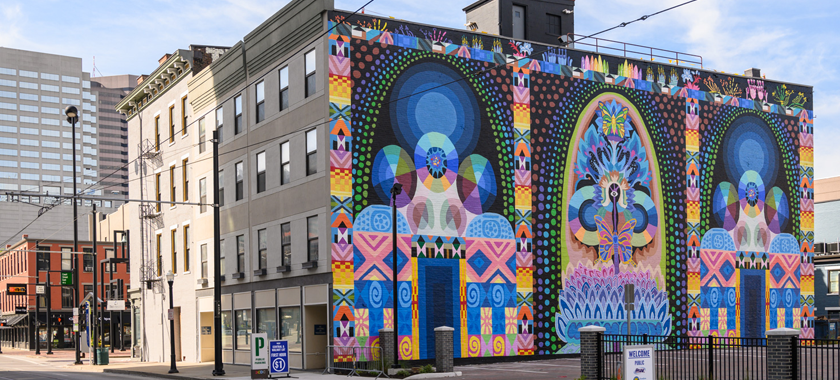This color photograph captures a vivid street scene framed by a beautiful blue sky. Dominating the foreground is a black metal fence along the sidewalk, featuring a "Welcome Park" sign. Just behind the fence stands a striking, three-story gray building adorned with ornate and colorful decorations. The building's wall boasts a series of three arches, with each arch filled with multicolored boxes and swirls in vibrant shades of pink, yellow, blue, and green. The arches themselves are intricately painted in circles of purple, blue, aqua, green, and yellow, making the façade particularly eye-catching.

The photo is taken at an angle that reveals both the front and side views of this gray building. While its front is a plain tan façade extending across much of the block, the intricate side view is what draws attention. Opposite this building, across the street, is a smaller, red-orange building with fewer floors. Further down the street, another taller building, similar in color to the tan front façade, is partially visible. Supplementing the urban atmosphere, a slew of utility poles and wires crisscross the scene, accompanied by a couple of streetlights. A small red light near the street corner hints at a pedestrian crossing or traffic light, while a parking symbol marked with a "P" provides additional cityscape details.